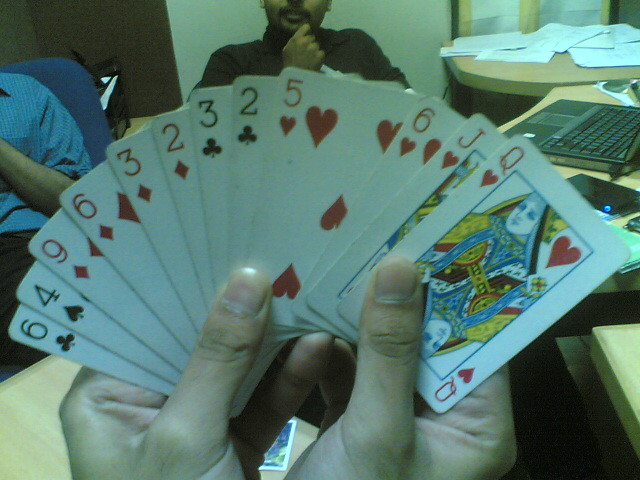In the foreground of the image, a person's hand holds up a fan of playing cards. The cards, small and rectangular, are spread out to reveal their intricate designs and suits. Dominating the scene is the Queen of Hearts, a card with a white background and a detailed blue rectangle at its center. The queen is depicted wearing a yellow hood and an elaborate yellow and blue dress. Her image is mirrored; her face is at the top and inverted at the bottom. The card's corner features a bold "Q" and a heart symbol. Peeking from behind this queen are other cards, including a Jack of Hearts, a Six of Hearts, a Five of Hearts, a Two of Clubs, a Three of Clubs, a Two of Diamonds, a Three of Diamonds, a Six of Diamonds, a Nine of Diamonds, a Four of Spades, and a Six of Clubs. Each card is carefully held in place by the person's thumbs.

In the blurred background, the setting appears to be a busy office or a communal workspace. There are several desks cluttered with laptops, messy papers, and other office paraphernalia. Slightly obstructed by the cards, a man is partially visible, adding a sense of human presence. Off to the side, another person's shoulder and arm can be seen, suggesting a room filled with activity and workers engaged in various tasks.